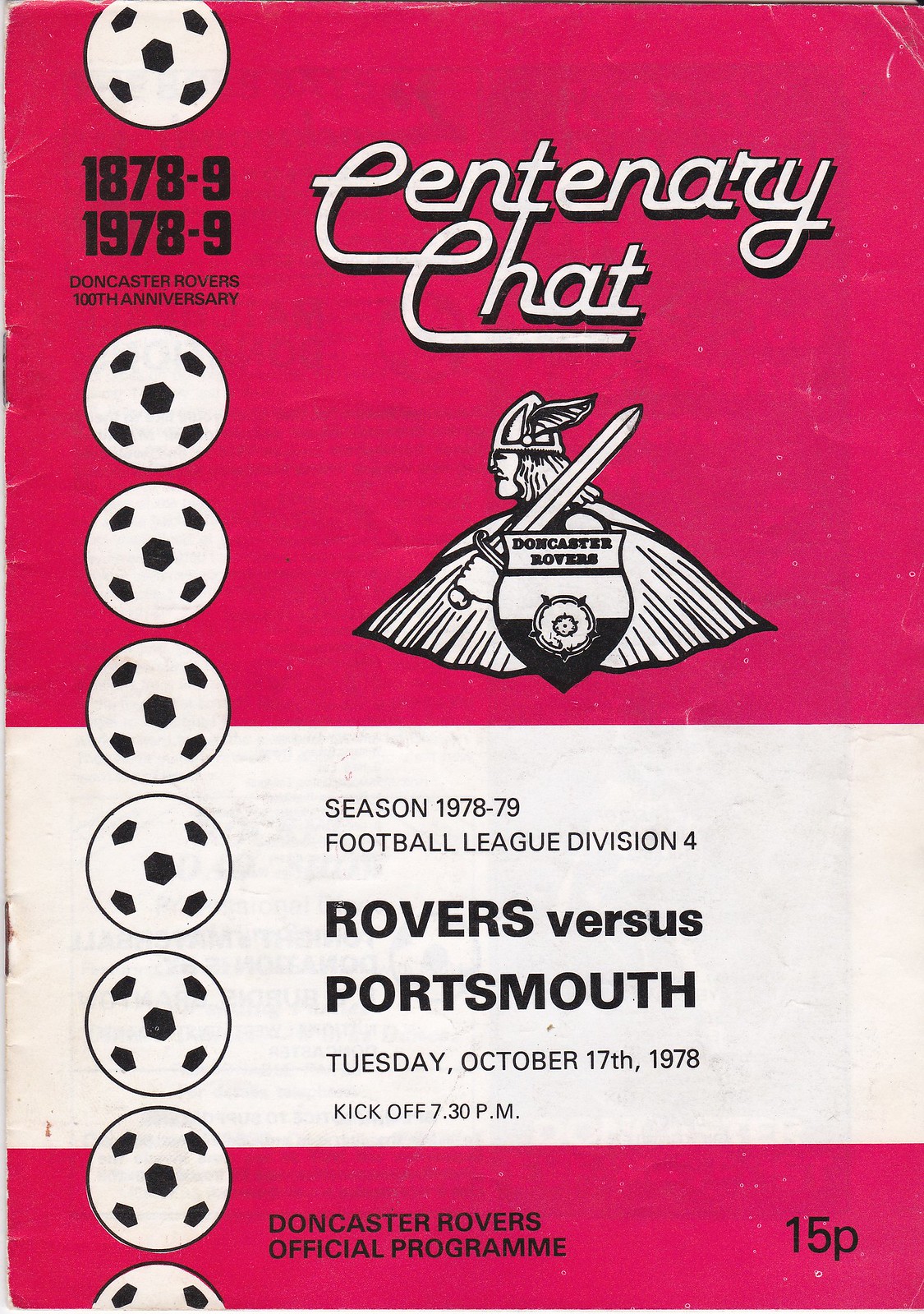This image depicts the front cover of an official football program, most likely from a European league given the use of the term "football" which references soccer in Europe. The program dates back to the late 1970s, specifically covering the years 1978-79. The cover features a prominently displayed football (soccer ball), further indicating its European origins. It appears to be aged, with what was likely originally white now faded to a tan color. The typography is notable, with a mix of bold and century chat fonts adding to the vintage charm. Additionally, the cover incorporates the team's mascot and various icons related to the sport. The overall color scheme is basic, dominated by red, adding to its classic feel. The program provides a fascinating glimpse into sports history from that era.